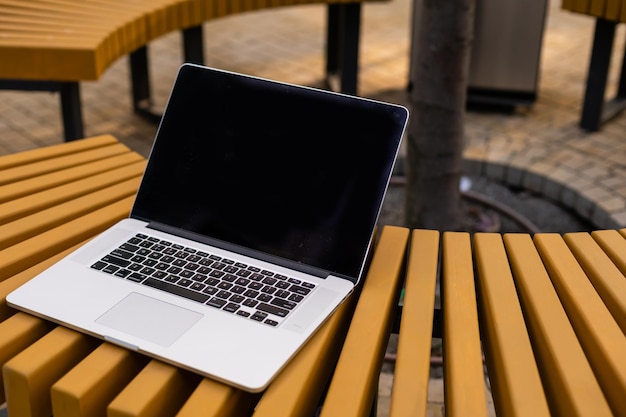A sleek silver laptop with a black screen and matching black keys rests on an unconventional yellow bench. The bench, made from thin, square-shaped slats, encircles a tree, of which only a fragment of the trunk is visible. The unique seating is positioned against a backdrop of charming cobblestone streets, adding a rustic touch to the modern scene.